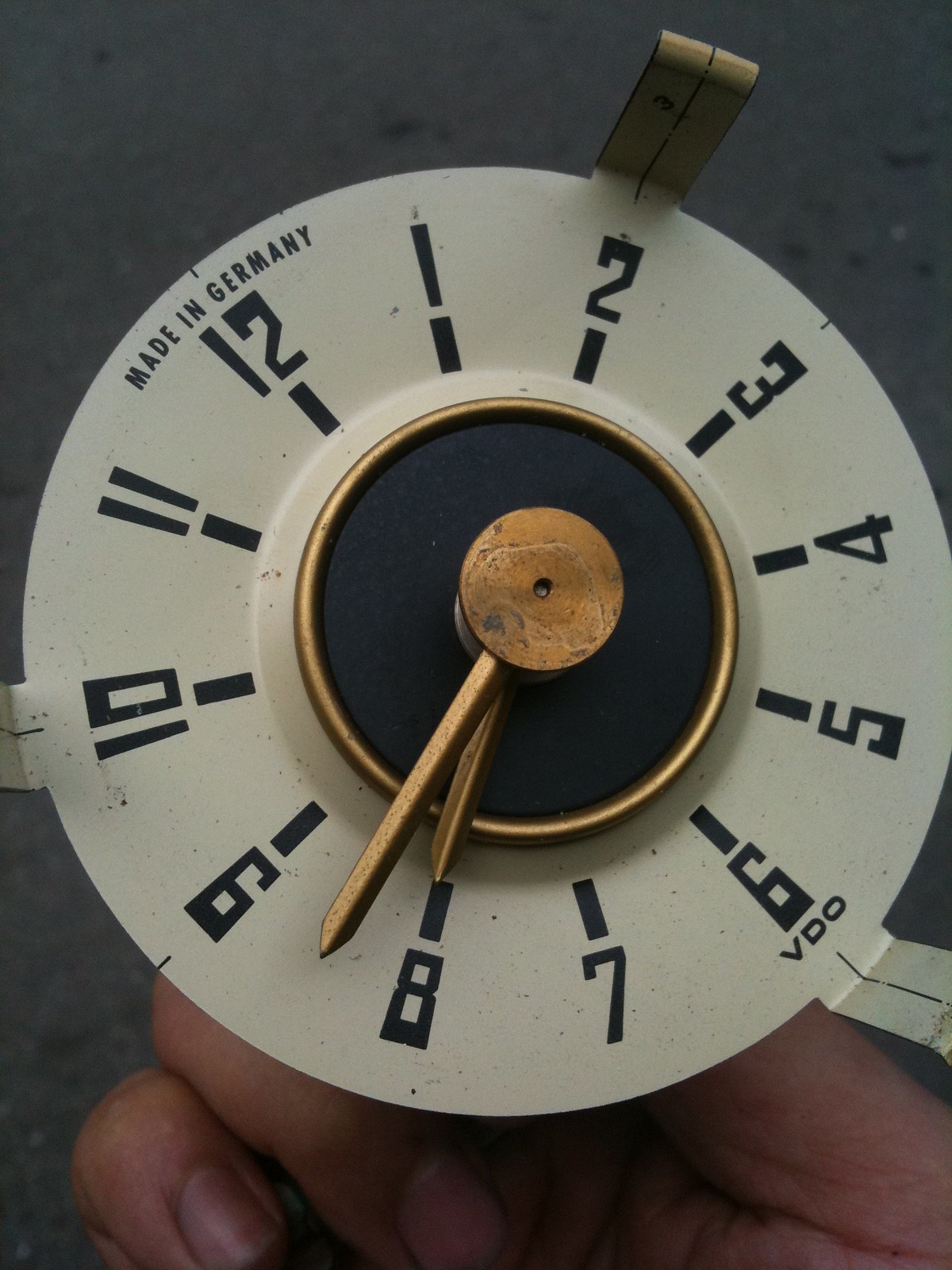This photograph captures a close-up of a white clock face, held indoors under dim overhead lighting. The bottom portion of the image is dominated by a partially visible right hand, likely gripping the clock between the forefinger and thumb in a palm-up orientation. The background is a dark grey surface, enhancing the contrast with the clock's light color.

The clock face is detailed with distinctive markings: positioned above the 12 o'clock numeral, the text "Made in Germany" is prominently displayed. Below the 6 o'clock numeral, the brand name "VDO" is inscribed. The numerals themselves are styled in a retro, early computer font, adding a sense of vintage charm to the timepiece.

At the center of the clock face is a raised black circle, surrounded by a brass-colored ring. The central mounting piece is also brass-colored, providing a cohesive look with the two hands, which share the same metallic finish. The minute and hour hands are elegantly designed, completing the sophisticated and timeless appeal of the clock.